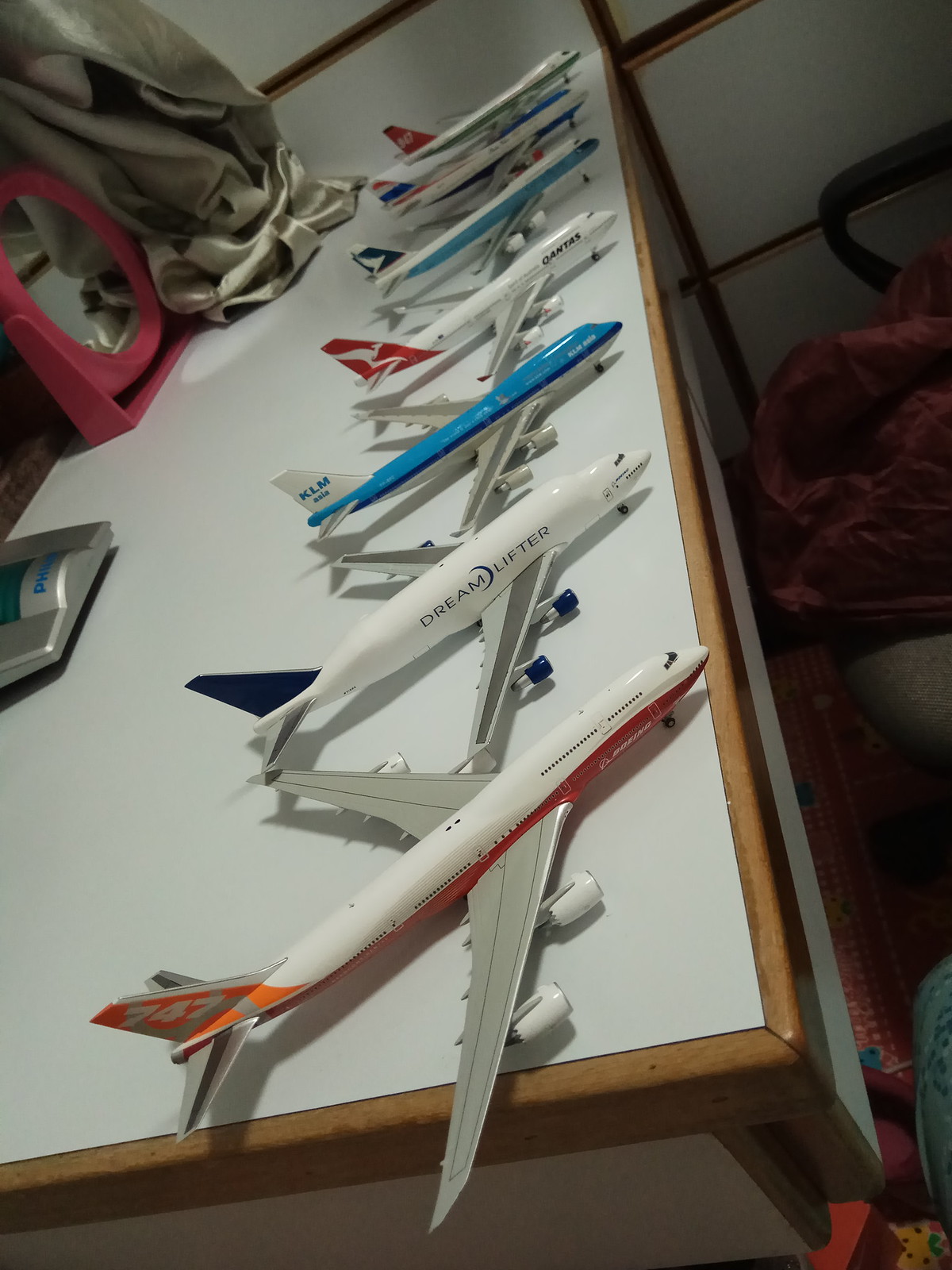The image depicts an indoor scene centered on a sleek desk with a brown wooden frame and a white inset top, laid out at an angle in the photograph. Positioned neatly across the right-hand edge of the desk are seven miniature model airplanes. Each plane is primarily white, but they feature distinct touches of blue, red, and orange accents. The closest plane has a white and red design, while another model, labeled with "Dream Lifter" in blue text, stands out among the line-up. Behind these planes, the back edge of the desk is adorned with a small pink round mirror and what appears to be a silverish fabric or robe hanging from the top left corner. Additionally, a part of a telephone is visible, suggesting this is likely a workspace or hobby area in someone's room. The model planes appear to be assembled kits, organized meticulously as decorative items on the smooth, polished surface of the desk.